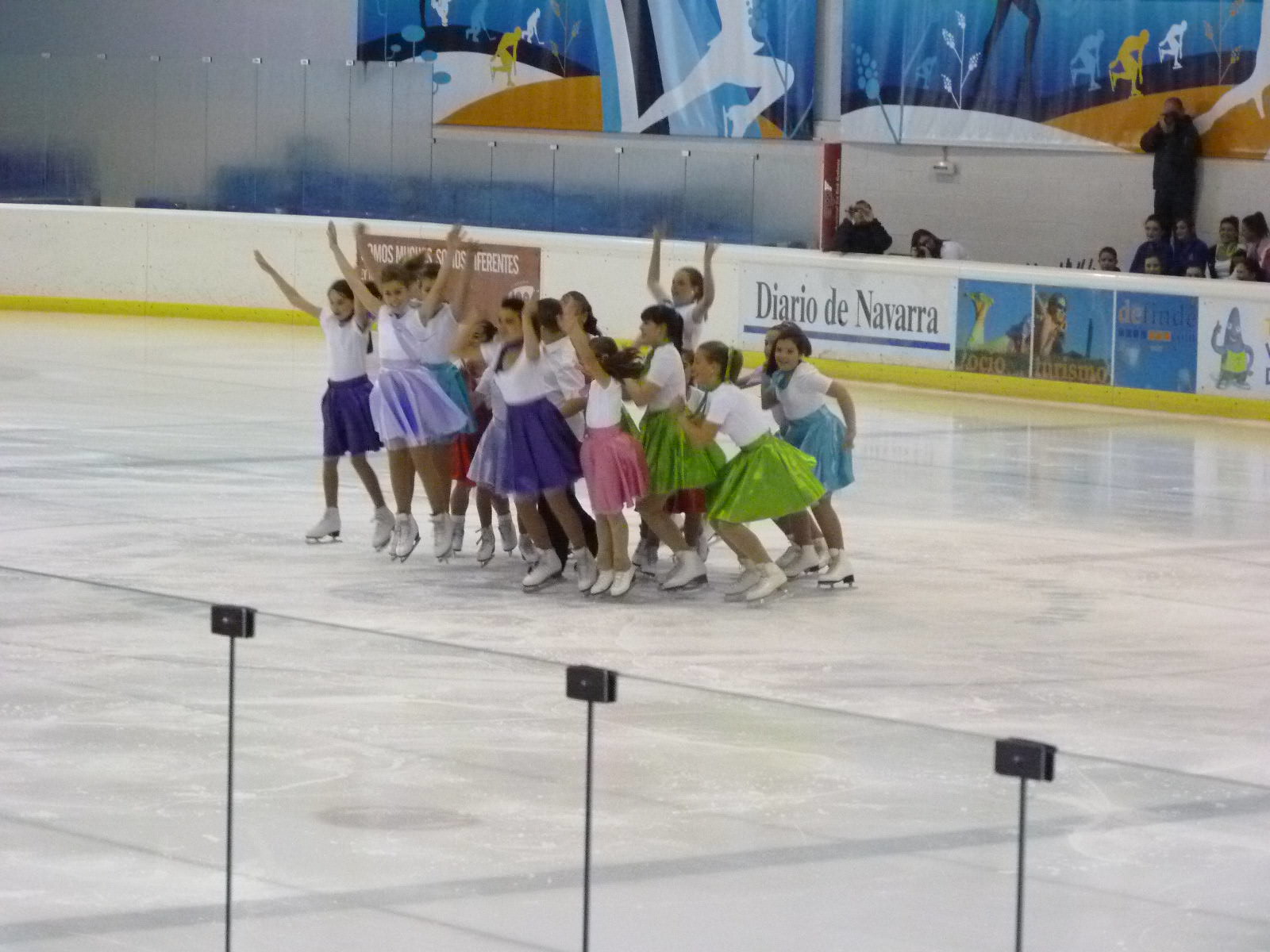An indoor color photograph captures a lively moment at an ice rink, where a group of young, enthusiastic ice skaters, all approximately 10 to 21 years old, are performing what appears to be the finale of their show. Dressed in white tops and a mix of vibrant skirts reminiscent of the 50s and 60s—featuring colors such as purple, lavender, blue, pink, and green—the skaters, around 13 or 14 in number, are seen in various stages of a jubilant jump. Their arms are raised high, seemingly cheering or exclaiming something in unison. The rink's glass protection barrier is visible in the foreground, while the background features a wall adorned with posters, signs, and a mural depicting dancers. Beyond the mural, spectators and families eagerly watch and capture the moment. The wall in the background also displays some text in Spanish, suggesting the location might be in Spain, with mentions of "Diario de Navarra" and "Ocio Turismo." Despite being slightly out of focus, the photograph vividly conveys the excitement and energy of this ice skating performance.